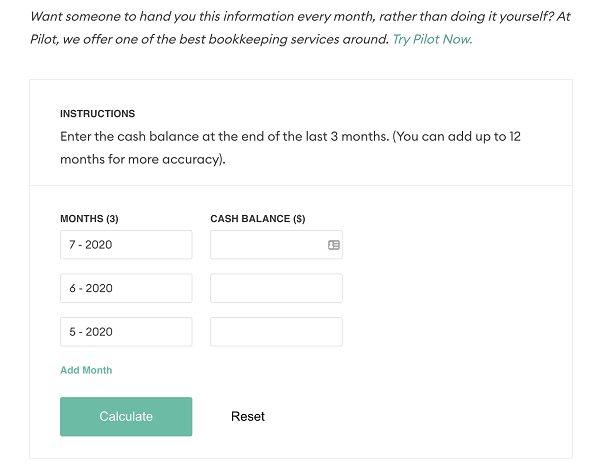An informative screen displays a financial data entry form for Pilot's bookkeeping service. At the top, there is promotional text in bold, inviting users to offload their monthly bookkeeping tasks to Pilot: "Want someone to undo this information every month rather than doing it yourself? At Pilot, we offer one of the best bookkeeping services around. Try Pilot now." Below this, the screen provides specific instructions: "Enter the cash balance at the end of the last three months. You can add up to 12 months for more accuracy."

The interface includes several elements for user interaction. Three horizontal bars with dates "5/20/2020," "6/20/2020," and "7/20/2020" allow users to input their cash balances. There is also a dynamic green text option to "Add Month" if more months need to be included. At the center, a prominent green rectangle labeled "Calculate" invites users to process their entries. Additionally, a "Reset" option is available to clear the inputs.

The screen features a clean design with white borders and gridlines, which help to separate and organize the different interactive sections.